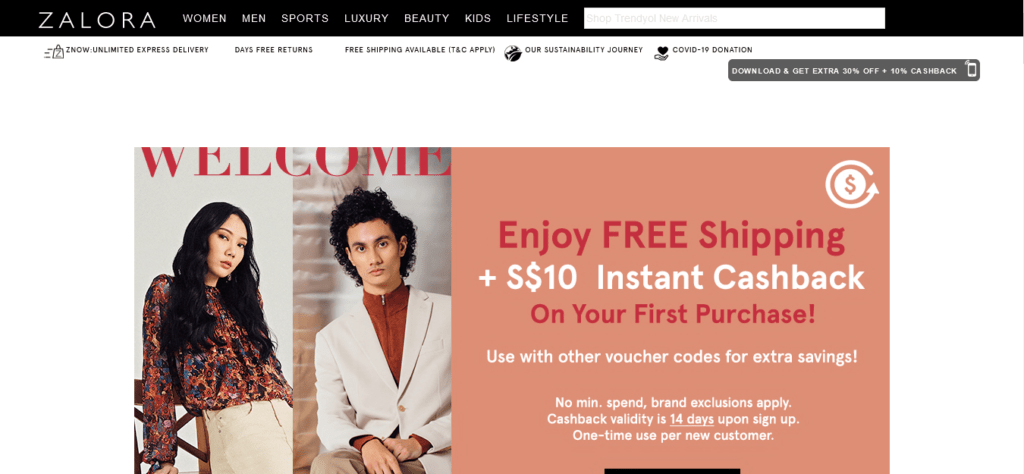The image displays a website with a sleek, modern interface. At the top is a black banner featuring the site's logo, "Zalora" in bold white letters. Adjacent to the logo, there's a horizontal menu bar with categories such as Women, Men, Sports, Luxury, Beauty, Kids, and Lifestyle. Directly beneath this menu is a white search bar labeled "Shop Trendy New Arrivals."

As your eyes move downward, the background transitions to white, where promotional text highlights various perks: "Now Unlimited Express Delivery," "30 Days Free Returns," and "Free Shipping Available," with a note in parentheses that reads "(TNC apply)." Additional messages on sustainability and COVID-19 donation efforts follow.

Next, a gray banner with white text encourages mobile app downloads, offering "Extra 30% Off Plus 10% Cashback" with an accompanying graphic of a smartphone.

Further down, a rectangular section is divided into two parts. On the left, a welcoming message above images of a man and a woman reads, "Welcome." The right side, featuring a peach and melon background, prominently displays in reddish-pink text, "Enjoy FREE Shipping," and in white text, "$10 Instant Cashback" on the first purchase. Below this, additional white text states, "Use with other voucher codes for extra savings!" and "No min spend, brand exclusion apply." The cashback's validity is underscored: "14 days (14 is underlined) upon sign-up. One-time use per new customer."

This captivating and informative layout highlights the website's offerings and promotions effectively.